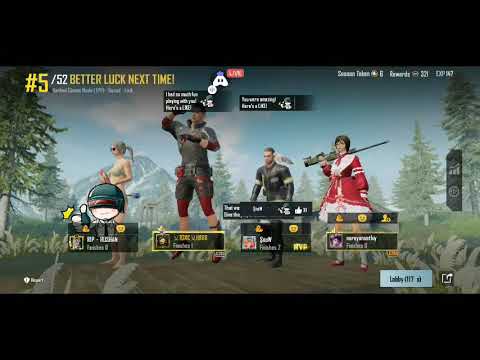The image appears to be a detailed screenshot from a video game featuring four distinct characters in unique costumes, standing outdoors on rocky terrain with a scenic backdrop of pine trees, mountains, and a bright blue sky scattered with puffy white clouds. Positioned from left to right: the first character is a woman adorned in a small top resembling a bra, paired with shorts, and accessorized with sunglasses, gray hair styled in a ponytail, and is turned slightly away from the camera. Adjacent to her stands an athletic man in tight red shorts, a gray shirt with a large collar, and red gloves, striking an action pose with one hand raised. The third character, positioned slightly towards the background, is a man dressed in a black body suit accentuated with white armbands. The final character is a woman clad in a red dress with white flared edges, reminiscent of a Christmas outfit, holding a sniper rifle over her shoulders and donned with red-heeled footwear. Overlaying the characters are various game stats and character attributes. In the top left corner, the overlay shows "5/52" and the message "better luck next time," accompanied by a small discord symbol.